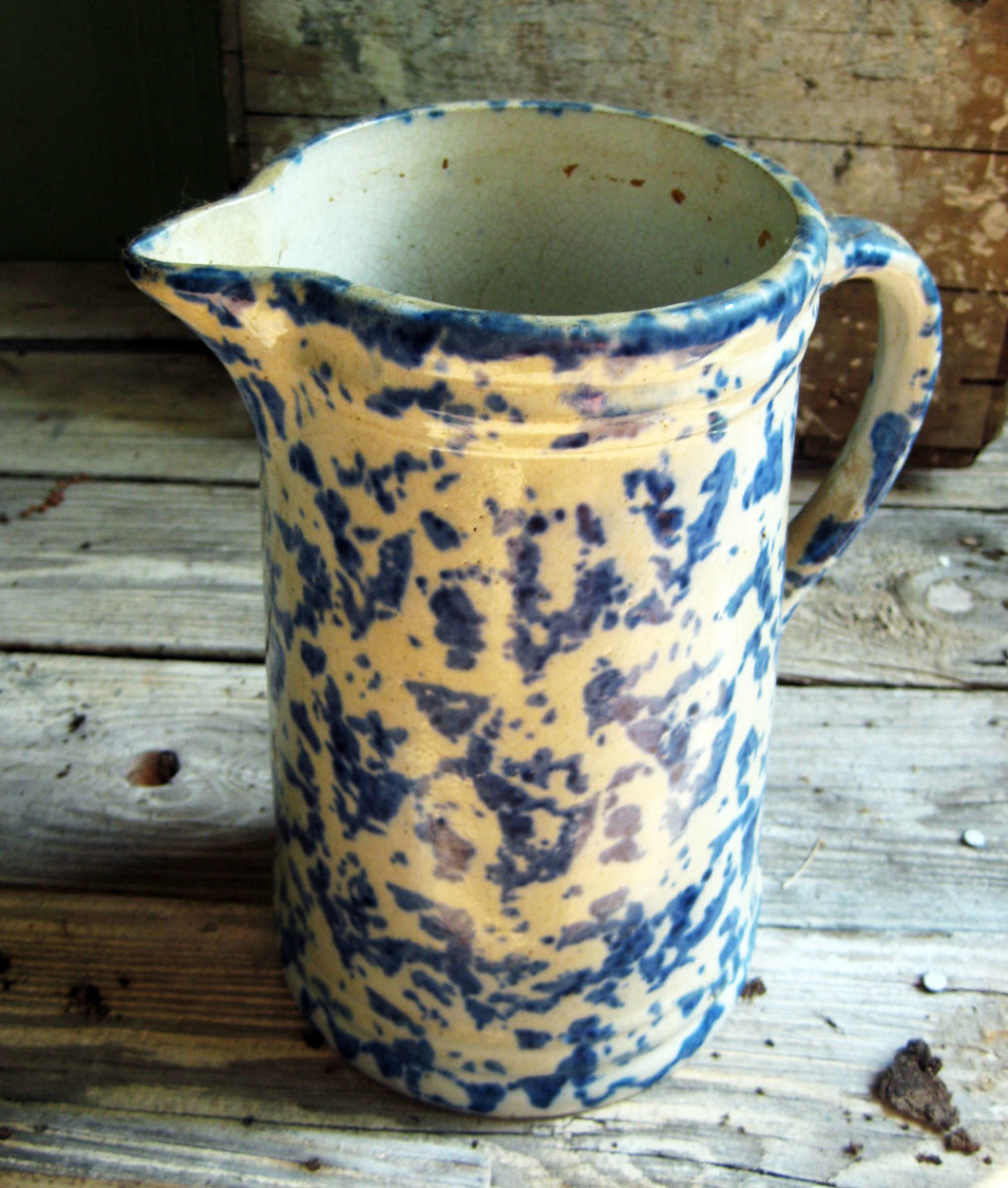This photograph showcases an antique ceramic pitcher, primarily yellow with blue splotches creating a unique pattern. The pitcher, with its handle on the right and spout on the left, is positioned prominently on weathered wooden planks, suggesting an old porch or rustic floor. The distressed wood, full of imperfections like nail heads and holes, enhances the vintage feel of the image. Additional elements like a clump of dirt near the pitcher contribute to the rustic ambiance. Behind the pitcher, there's a similarly worn-out wooden wall, further emphasizing the aged setting. The inside of the pitcher appears cream-colored, and no liquid is visible within. The overall composition highlights the pitcher as the focal point, with its vivid colors standing out against the muted, earthy tones of the background.